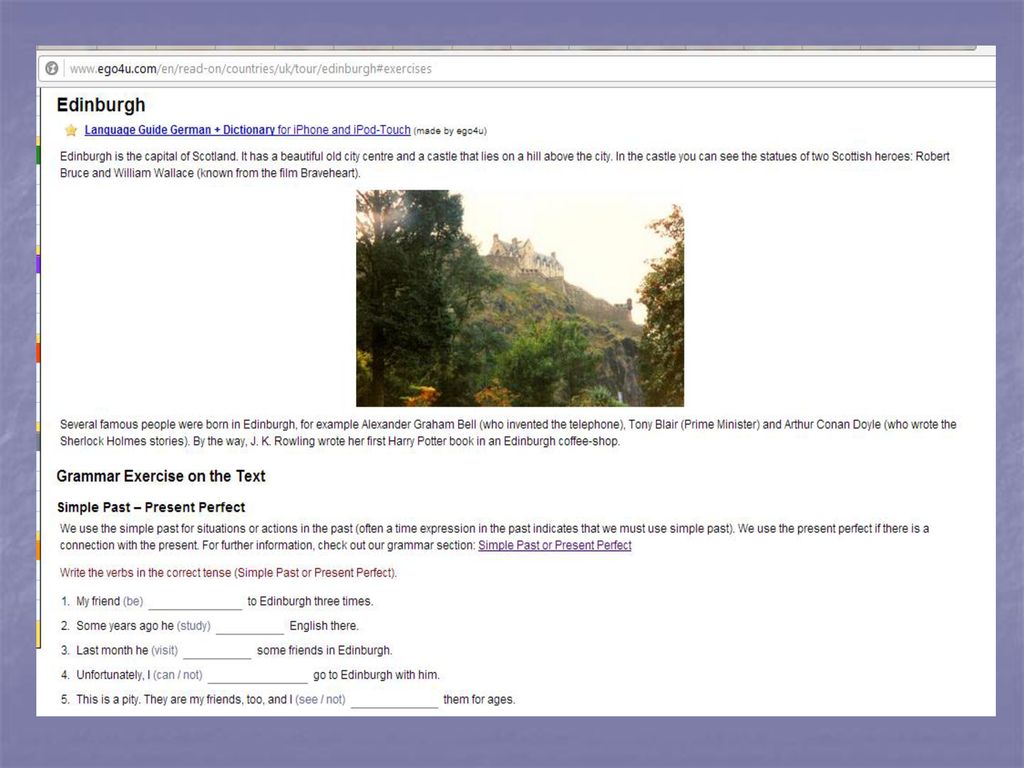**Caption:**

The image showcases an informative web page with distinct visual elements and educational content. The central area of the page is a white rectangle bordered in purple, with a noticeable gray circle at the top containing a shape resembling a cat. The browser is highly zoomed in, which causes some parts of the webpage to be cut off. 

At the top, the URL is displayed in gray as "www." followed by "egoforyou.com" in black. Below this, the word "Edinburgh" is prominently written in black, accompanied by a yellow star. The text "Edinburgh" is set on a purplish background. The following information is listed in purple: "English Guide German, Play Stationary for iPhone, and iPod Touch."

Further down, in black text, it states: "Made by Ego4U. This is Edinburgh. Edinburgh is the capital of Scotland. It is renowned for its beautiful old city center and the iconic castle that stands on the hill overlooking the city. Within the castle, visitors can see statues of two Scottish heroes, Robert Bruce and William Wallace, who are also featured in the film Braveheart."

Below this, there is an image of the Edinburgh Castle surrounded by lush green trees, emphasizing its elevated position. The text continues in black: "Several famous people were born in Edinburgh, such as Alexander Graham Bell, the inventor of the telephone, Tony Blair, a former Prime Minister, and Arthur Conan Doyle, the author of the Sherlock Holmes stories. Additionally, J.K. Rowling wrote her first Harry Potter book in an Edinburgh coffee shop."

Towards the bottom, the web page provides a grammar exercise titled "Grammar Exercise on the text, Simple Past to Present Perfect." It explains: "We use the simple past for situations or actions that happened in the past, while we use the present perfect if there is a connection with the present. For further information, check out our Grammar section, Simple Past to Present Perfect."

This detailed caption captures both the visual layout and comprehensive educational content of the webpage.